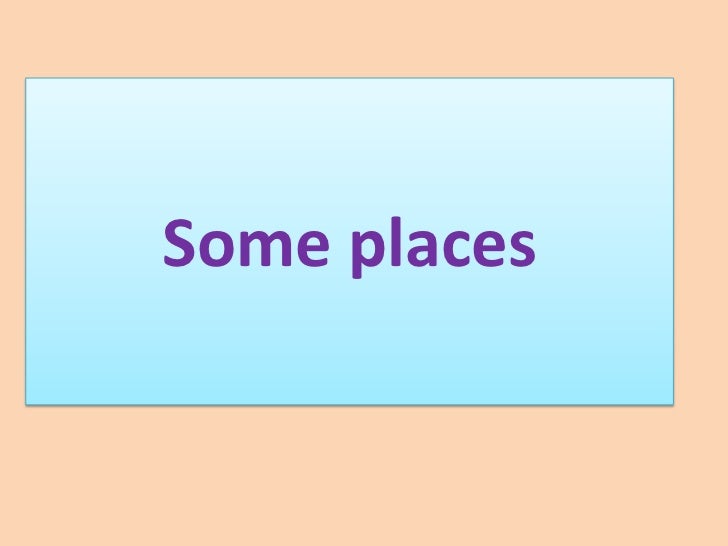The image features a large, rectangular background with a peach to light orange-pink gradient. Slightly off-center and positioned closer to the top and left side, there is a long rectangle with a light blue gradient that transitions from white at the top to a deeper light blue at the bottom. This blue rectangle has a dark blue outline. In the center of the blue rectangle, in bold purple text, it says "Some Places," with the “S” in "Some" capitalized and a space between the two words. The purple lettering is centrally aligned within the blue rectangle against the contrasting background. There are no other elements or details in the image.